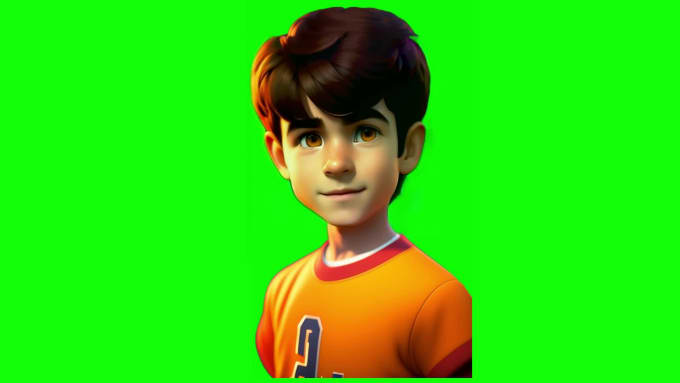The image depicts a 3D computer-generated small Caucasian boy with a cartoonish appearance, set against a neon green background. The boy has short, slightly tousled brown hair with swooping bangs, light brown eyes, and big eyebrows. His face is fair-skinned, and he has a gentle smile. He appears to be wearing an orange jersey with a red collar and possibly a white undershirt beneath it. The shirt seems to have some kind of blue detailing down the center, though it is partially cut off as the image only shows him from the chest upwards. The background is a vivid lime green, occupying most of the image, with no additional text or elements.